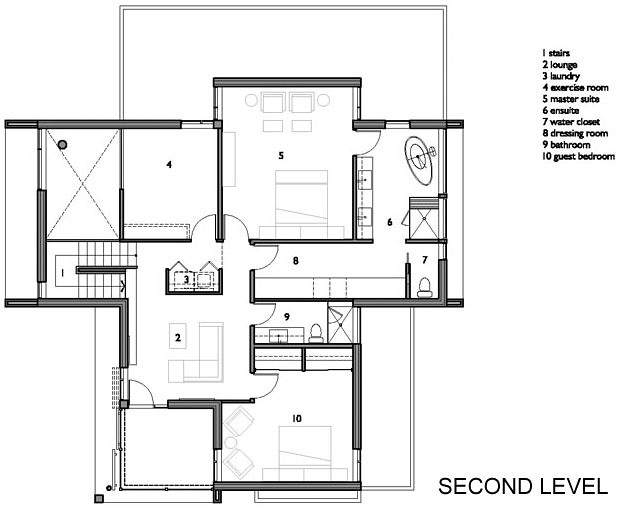This detailed blueprint of a residential home's second level is presented in a rectangular format with the top and bottom edges extending longer than the left and right edges. The entire image is rendered in primary shades of black and white, offering a clear and professional layout. In the bottom right corner, "SECOND LEVEL" is prominently displayed in bold, uppercase black text.

In the top right corner, there is an essential numbered legend that deciphers the various numbered rooms and areas marked throughout the blueprint. The legend reads:

1. Stairs
2. Lounges
3. Laundry
4. Exercise Room
5. Master Suite
6. End Suites
7. Water Closet
8. Dressing Room
9. Bathroom
10. Guest Bedroom

The outer walls of the second level are depicted with thick gray lines bordered in black, providing a solid structural outline. Doorways are detailed with thin gray lines accompanied by a curved indicator, which demonstrates the directional swing of each door.

In the bottom right corner of the blueprint, a large bedroom is illustrated, complete with light gray outlines of the furniture, giving a sense of space and layout within the room. Meanwhile, the top right corner houses the informative numbered table, ensuring easy reference and helping visualize the component parts of this thoughtfully designed living space.